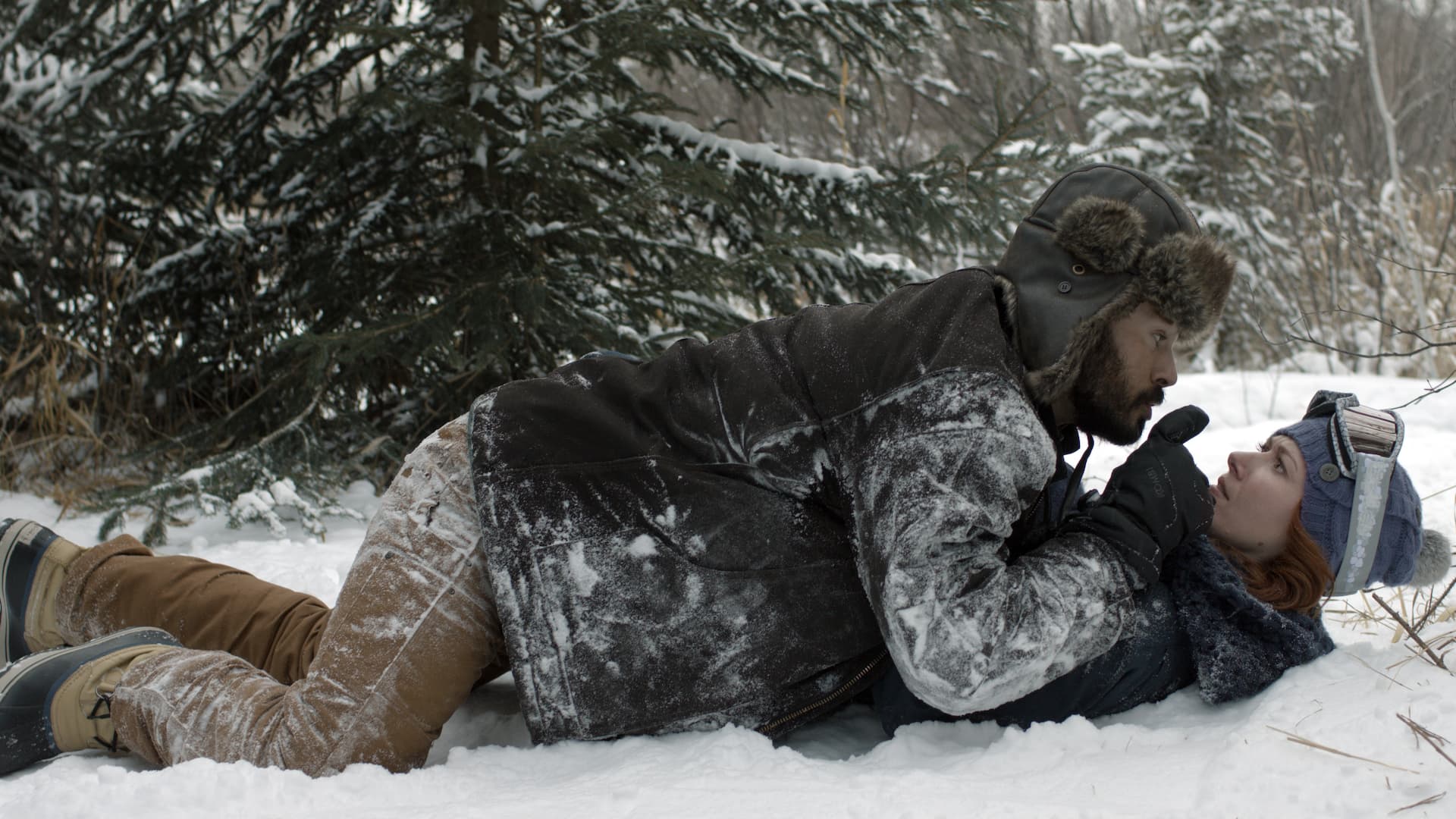Amidst a snowy, wooded landscape filled with evergreen trees dusted in white, a tense scene unfolds between a man and a woman lying on the ground. The man, a young Black man with a black beard and piercing gaze, wears a dark brown, ear-flap hat, a black jacket covered with snow, brown pants, and black boots. He leans over the woman, his stern expression accompanied by his gloved hand, finger pointed upwards, suggesting a warning or a need for silence. The woman, a white woman with red hair peeking out from under her blue beanie and white ski goggles perched on her forehead, lies mostly obscured by the man, her face displaying concern and confusion. Their winter clothes, dusted with snow, hint at a struggle in the icy environment. In the background, fir trees and some brown and yellow vegetation contribute to the stark, wintry setting, completing the dramatic and intense atmosphere.